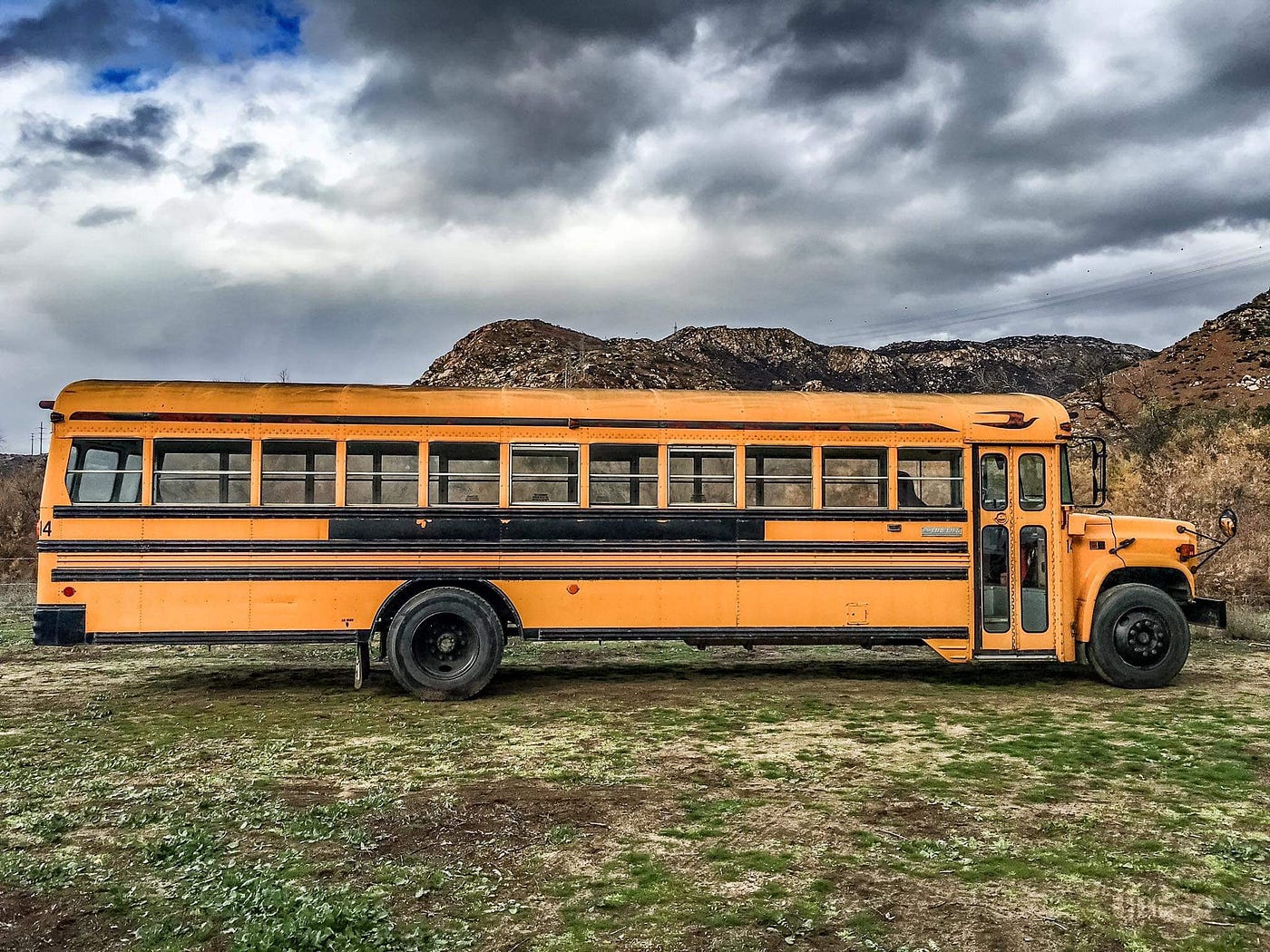This detailed image showcases a standard orange-yellow school bus, its paint now appearing dirty and faded, positioned centrally but slightly off to the left in a dry and semi-arid landscape. The bus, facing right with its rear to the left of the frame, occupies roughly a quarter of the image. Characteristic of a typical school bus, it features black tires, visible windows, and large double doors on the right side for student entry and exit. The first window reveals the bus driver’s seat, while the remaining windows vary between being open and closed, hinting at a possible conversion project. The bus lacks any identifying school district markings, with the area where such a name would appear either painted over or blacked out.

In the foreground, brown dirt interspersed with clumps of green grass is visible, contributing to the image's arid atmosphere. The backdrop is adorned with rolling hills, lightly dusted with dirt and sparse vegetation, stretching to a beautiful, albeit mostly cloudy sky. Dark gray and white clouds dominate the scene with a touch of blue peeking through the upper left corner, adding contrast to the otherwise monochromatic palette. The overall scene is one of quiet isolation, captured in an environment where nature and a relic of transportation quietly coexist.